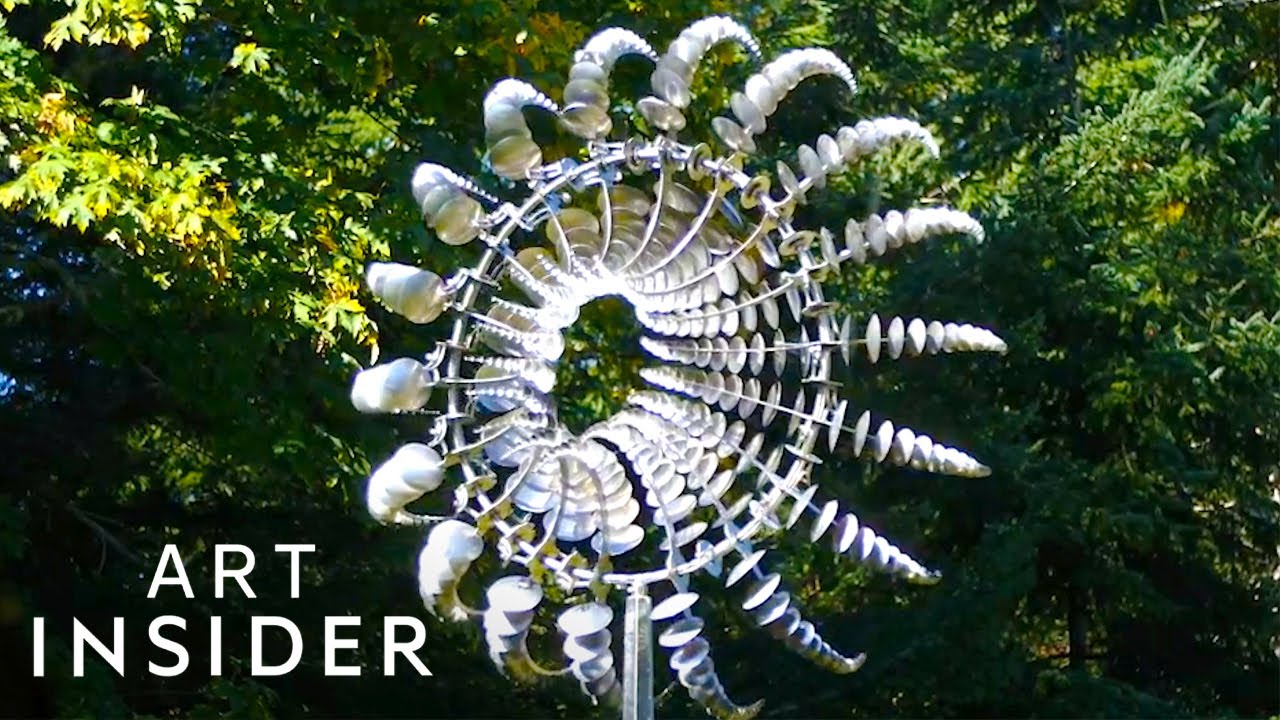This horizontal, rectangular photograph features an outdoor installation captured for "Art Insider," as indicated by the large, bold, white lettering in the lower left-hand corner. The centerpiece of the image is a striking, metal sculpture that resembles a sun motif, featuring a circular design with intricate leaf-like patterns and an empty center. The artwork appears to be mounted on a pole and is secured with a base for stability. Surrounding the sculpture are dense, dark green trees, creating a lush natural background. On the left side of the image, a shaft of sunlight pierces through the leaves, illuminating them and adding a dynamic quality that suggests movement, as if they are being blown by the wind. The darker lower portion of the scene contrasts sharply, allowing the sunlight and the intricate details of the sculpture to stand out prominently.